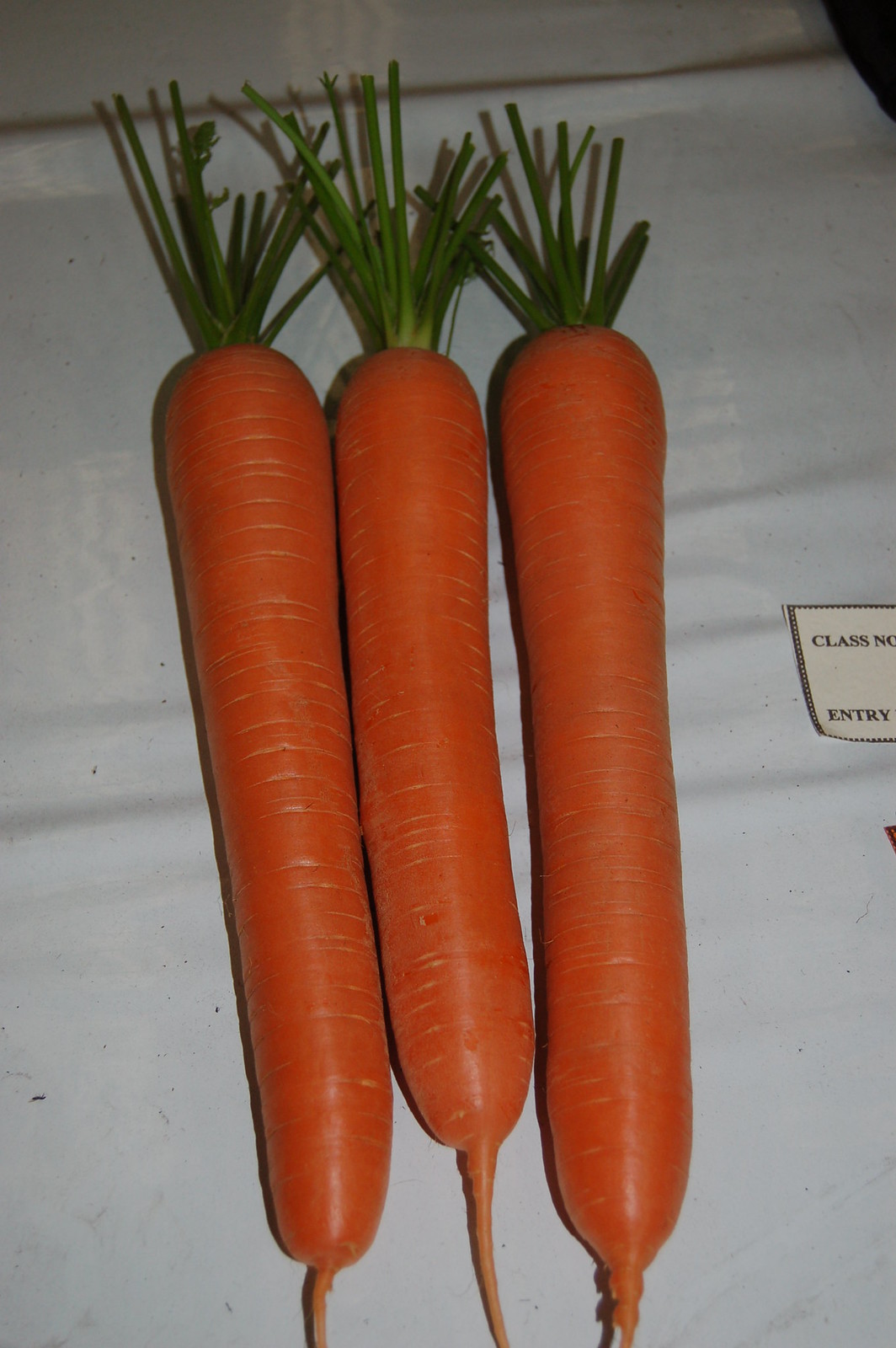This photograph captures three exceptionally bright and fresh-looking, chunky carrots arranged side-by-side in a vertical orientation on a white background, which could be cloth or wood. Each carrot has a shimmering orange hue with wrinkled divots and a bit of the bottom stem area attached. The tops of the carrots are adorned with trimmed sprigs of green stems, forming a small bouquet. To the right of the carrots, a partially visible card or label with black lettering can be seen, though the text is not entirely readable. The overall presentation suggests a careful arrangement, possibly for a vegetable competition, highlighting the impressive straightness and vibrant appeal of the carrots.